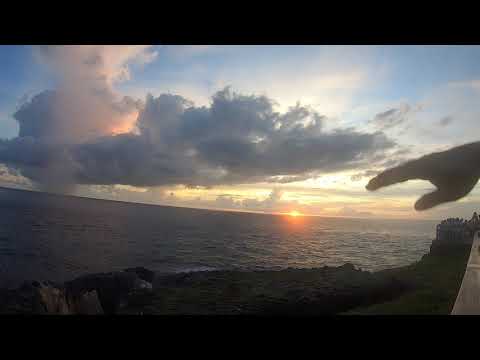The image captures a serene sunset over a calm body of water, possibly an ocean, viewed from a high vantage point. The horizon showcases an orange-pink sun receding into the distance, casting an ethereal glow over the slightly rippling waves. Large clouds, some dark and grouped together, hover above and around the sun, with the sunset’s pink light filtering through on the left. In the immediate foreground, a piece of rocky, green vegetation-covered land is visible but appears darkened, obscuring finer details. A right hand with fingers and thumb outstretched extends into the frame from the right side, seemingly gesturing toward the majestic sunset. The camera appears slightly tilted to the left, causing the horizon to slant gently down to the right by about 10 degrees.